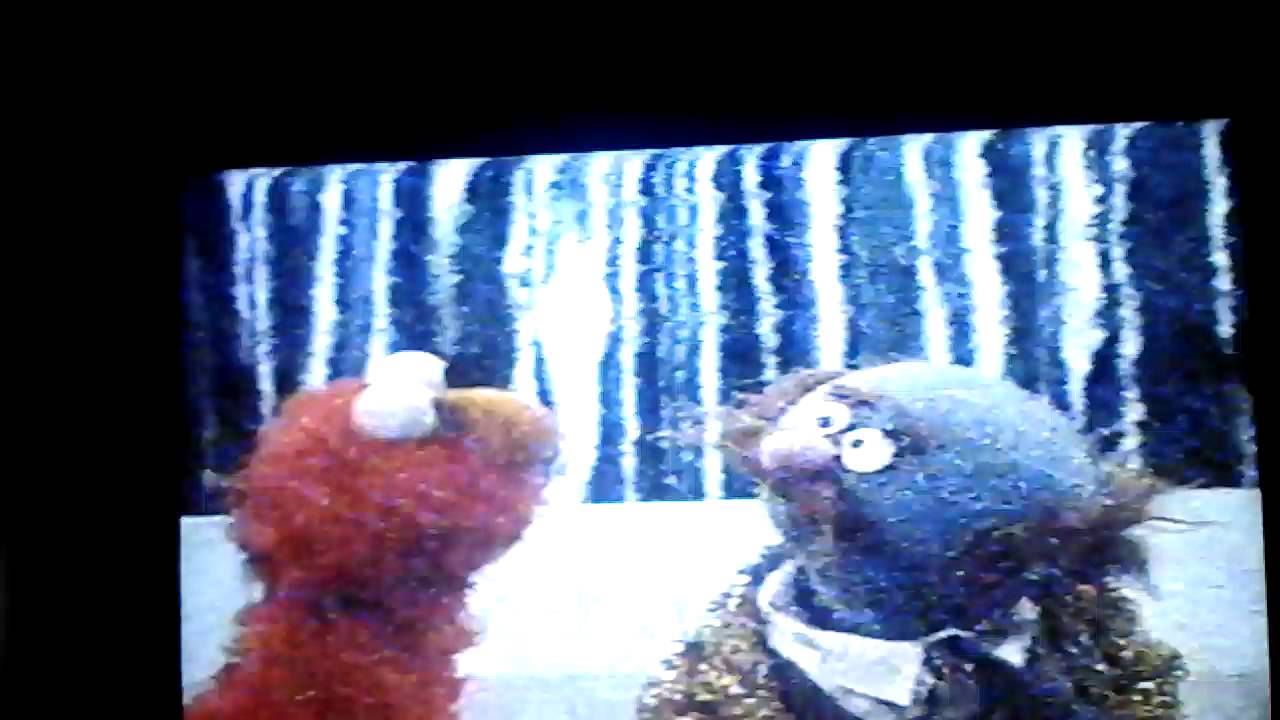In this detailed and somewhat skewed photograph of a TV screen, there are two Muppet characters prominently displayed against a predominantly black background. The character on the left is Elmo, identified by his iconic red fur and round white eyes perched atop his head. His head is slightly tilted as he faces right, engaging with the other Muppet. The second character, situated on the right, is a blue Muppet who appears to be an older figure, distinguished by his bald head with patches of hair on the sides. This character is dressed in a thick, greenish-brown sweater, suggesting a winter setting, further evidenced by snow on his jacket and a background scene that includes trees and snow. White vertical fuzzy lines appear in the background, possibly reflections or light. The depicted television screen occupies about three-quarters of the image and is framed unevenly with a thin black border on the right and a thicker black bar on the left. The image resolution is slightly grainy, contributing to a nostalgic, authentic feel of a candid television capture.